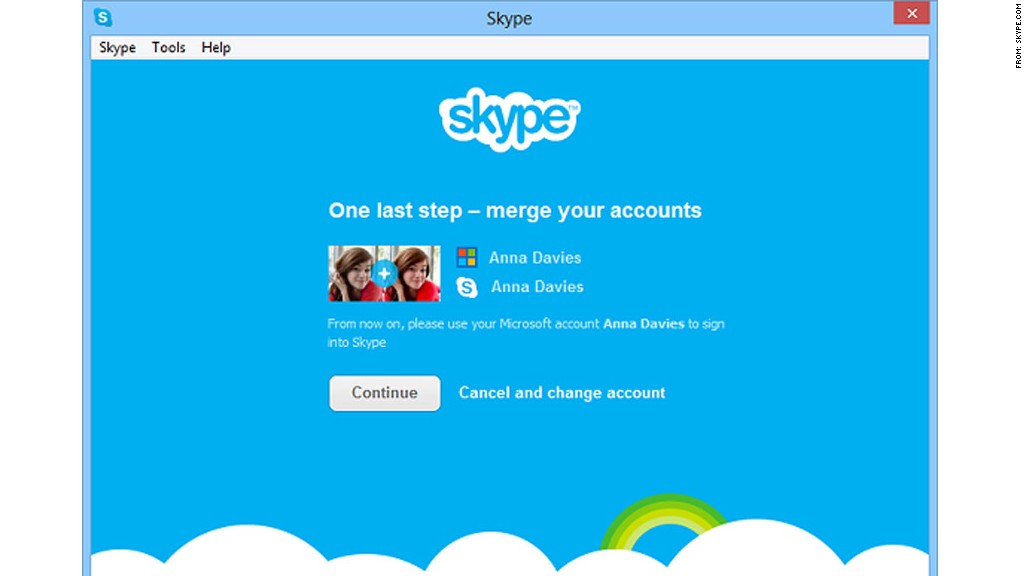The image depicts a Skype desktop application window prominently featuring a user interface with a dominant blue theme. At the top navigation bar, options for "Skype", "Tools", and "Help" are visible, offering additional functionalities upon clicking. A noticeable red exit button is positioned at the top right corner. 

The main section of the window showcases a serene sky-themed background, with a blue sky and fluffy white clouds, creating an impression of being above the clouds. Centrally placed is the classic Skype cloud logo with the word "Skype" embedded within it.

A notification in the foreground prompts the user to complete the final step of account merging. The message addresses Anna Davies, inviting her to merge her Microsoft and Skype accounts for streamlined access. Two profile pictures of a young white girl, presumably Ms. Davies, are displayed, symbolizing her existing accounts.

The message instructs the user to use their Microsoft account going forward and offers two interactive buttons at the bottom: a white "Continue" button to proceed with the merge, and a "Cancel and Change Account" option for those who may have reasons to opt-out.